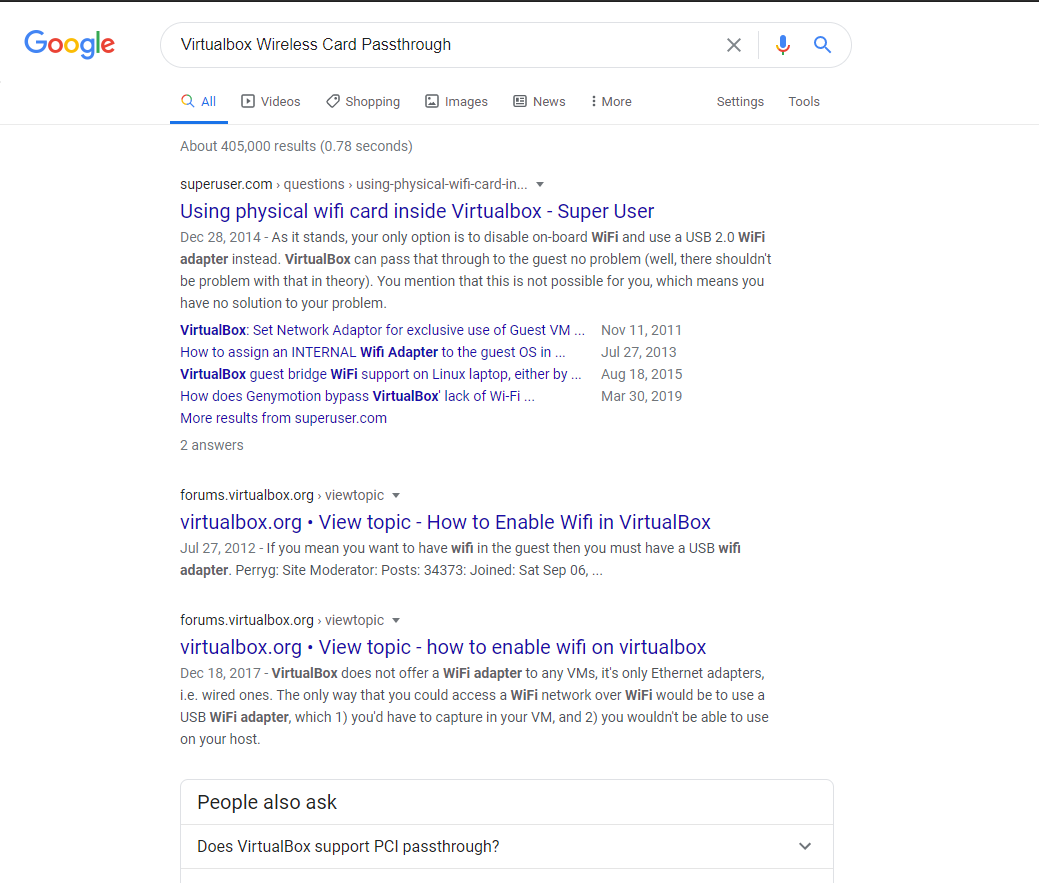A detailed description of the content in the provided image:

---

The image is a screenshot of a Google search results page dominated by a predominantly white background with black and blue text. At the top of the screenshot, there's a black horizontal band featuring the Google logo on the left and a search box in the center. The search query entered is "virtual box wireless card pass through."

Just below the search bar, various navigational tabs are visible, including "All," "Videos," "Shopping," "Images," "News," "More," and settings/tools that offer further search refinements. The "All" tab is currently selected.

Highlighted underneath these tabs is the search result summary, which states "About 405,000 results in 0.78 seconds."

The first search result is from Superuser.com, addressing a question posted on December 28, 2014, about using a physical Wi-Fi card within VirtualBox. The snippet of the discussion highlights the notion that, typically, the only feasible method is to disable the onboard Wi-Fi and use a USB 2.0 Wi-Fi adapter, which VirtualBox can pass through to the guest operating system without issues.

The second search result originates from the forums on VirtualBox.org, dated July 27, 2012. This thread elaborates on enabling Wi-Fi in VirtualBox, stipulating that a USB Wi-Fi adapter is necessary for Wi-Fi access within the guest.

The third result, also from VirtualBox.org's forums, posted on December 18, 2017, reinforces that VirtualBox does not natively offer a Wi-Fi adapter for virtual machines, only Ethernet (wired) adapters. This entry again suggests using a USB Wi-Fi adapter as the solution, which has its limitations concerning usability in both the host and virtual machine simultaneously.

Additionally, there is a section titled "People also ask" at the bottom of the search results, featuring common related queries. One visible question is, "Does VirtualBox support PCI passthrough?" This segment includes expandable answers revealed by clicking the downward arrows next to each query.

Overall, the search results focus on troubleshooting and understanding the constraints and solutions related to enabling Wi-Fi functionality within a VirtualBox environment.